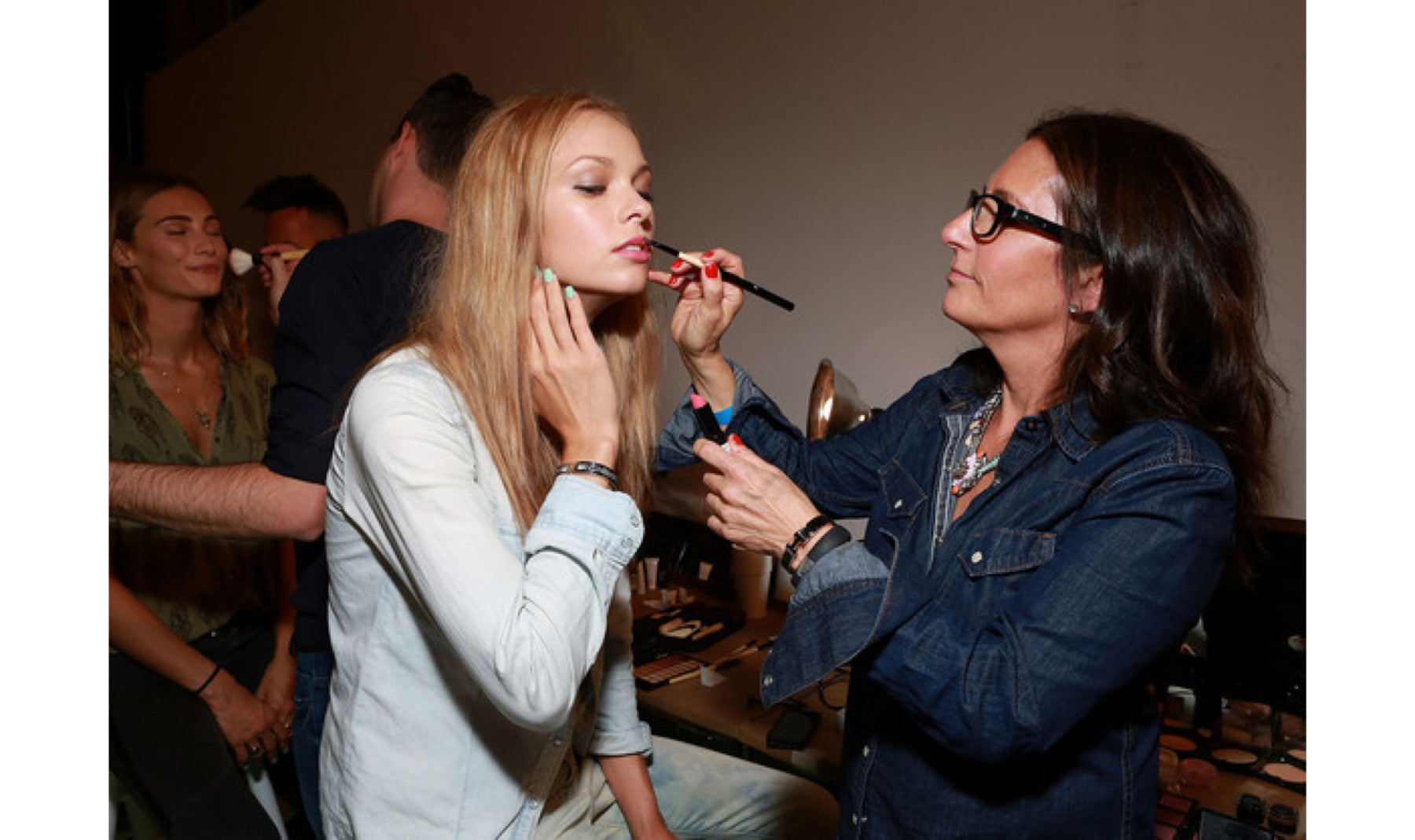In this close-up photograph, two women are centrally featured, with the background slightly out of focus, revealing other individuals receiving similar makeup treatments. The woman on the left, likely the model, has long, loosely flowing blondish hair extending past her waist and styled forward. Her fair skin contrasts with her light green nail polish. She’s dressed in a cream-colored denim jacket that complements her pink-colored lips, which are being carefully outlined by the woman on the right. This second woman, presumably the makeup artist, holds the makeup stick like a pencil and has tanned, slightly bronzed skin. She sports medium-length, wavy dark brown hair and wears black glasses along with a vibrant, multicolored necklace. Her attire includes a dark blue denim shirt, and her right-hand nails are painted red. In the blurred background, another woman in a green shirt receives makeup from a male artist, adding a dynamic backdrop to the detailed scene in the foreground.